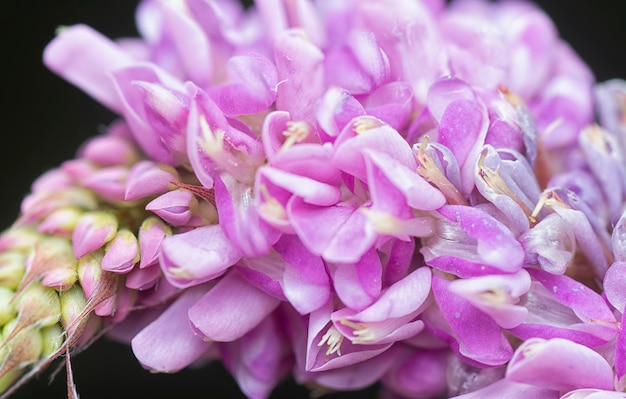The image is a small rectangular close-up color photograph featuring a prominent pink flower against a black background. The flower displays hundreds of small light purple petals in full bloom, showcasing numerous stamens and reproductive parts. Towards the left side of the flower, there's a green stem with less mature flowers that are still developing their pink color, resembling the top of a grass or wheat stalk. The matured flowers contrast beautifully with the tightly packed, greenish-yellow buds that are yet to bloom.